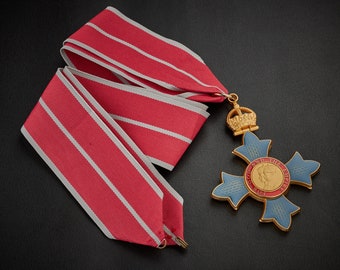This photograph presents a detailed, close-up view of a distinguished medal set against a black background. The medal, made of metal, features a blue cross with four leaf-like projections extending from the center in the cardinal directions. In the center of the cross, a circular design with a red rim and a gold core displays faces in profile. Crowning the top of the blue cross is a golden crown, which is linked to a loop that attaches to a broad ribbon, allowing the medal to be worn around the neck. The ribbon is predominantly red with white stripes along its edges and down the center, folded neatly on the left-hand side of the image, while the blue cross rests on the right-hand side. The scene is meticulously captured, highlighting the medal's intricate details and the ribbon's vibrant colors.